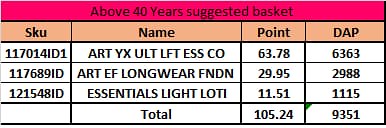The image depicts a small, horizontal, rectangular table resembling a screen capture from an Excel spreadsheet. The top row, with a dark pink background, is centered with black print reading "Above 40 Years Suggested Basket." This header is followed by four columns, each with a brown background and black text: "SKU," "Name," "Point," and "DAP." 

Under the SKU column, three identification numbers are listed: 1170141D1, 117689ID, and 121548ID. The corresponding names in the "Name" column are ArtYXALTLFTESSCO, Longwear Essentials, and Essentials Light. The "Point" column displays values in descending order: 63.78, 29.95, and 11.51. Finally, the "DAP" column includes numerical entries such as 6363, which accumulate to a total at the bottom of the table. This total sums up to a "Point" value of 105.24 and a "DAP" value of 9351, providing a comprehensive overview of the contents in a categorized format.